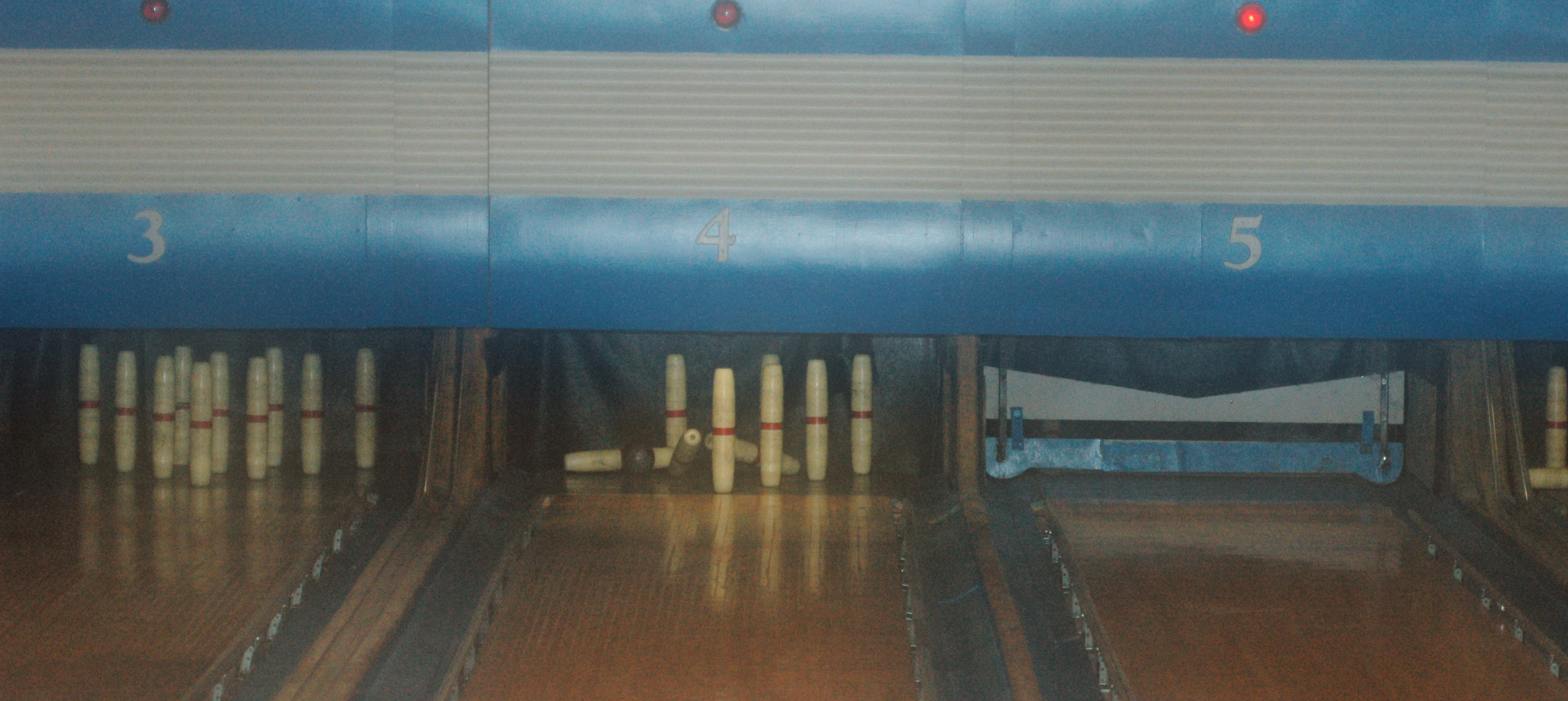The photograph captures the end of a bowling alley, focusing specifically on lanes 3, 4, and 5. Each lane is set against a striking blue upper wall accented with a gray streak and a series of small, illuminated round circles. The shiny wooden floors extend into the frame, including the gutters where stray balls might land.

Lane 3 features an entire set of unusually slender, cylindrical white pins with red trim, fully arranged in their classic triangular formation. Lane 4 shows a dynamic scene where a small bowling ball has just struck, knocking over several pins, while six pins remain standing, suggesting others may be obscured from view. 

Lane 5 is in reset mode. A mechanical arm is visible, sweeping away the fallen pins, and a warning red light above indicates the lane is temporarily closed. Additionally, a white and blue gate is lowered across the lane, possibly signaling it is out of service. A glimpse of lane 6 is also visible at the edge of the photo, hinting at the continuation of lanes beyond the captured frame. No people are present in the shot, focusing attention on the machinery and action at the end of the lanes.